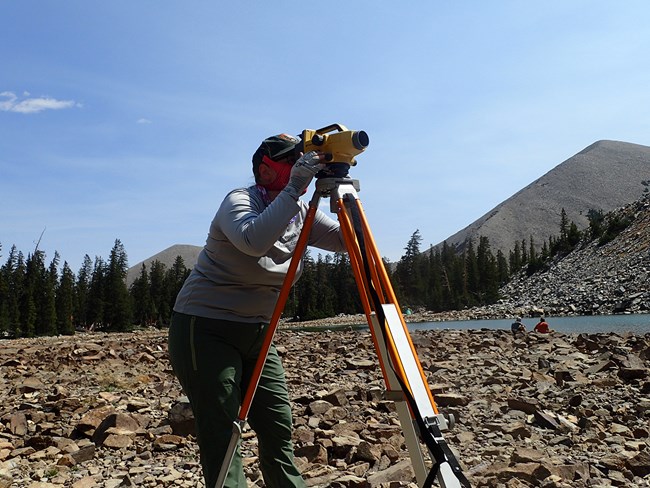In the photograph, a surveyor is meticulously focused on using a yellow and black surveying camera mounted on a silver and orange tripod. The surveyor is a woman, wearing a gray long-sleeve shirt, a blue cap with an emblem, green pants, gloves, and an orange face mask, blending diligently with her rocky surroundings. She stands in the middle of the frame, intently looking through the camera toward a mountain. The backdrop reveals a vast, rocky terrain dotted with brown rocks, transitioning into a lush landscape with green shrubbery and a small collection of evergreen trees. Behind her, there is a serene lake with two people sitting close to the water's edge, one wearing a gray shirt and a cap, and the other in a red shirt and cap. They are positioned near the water which reflects the natural beauty of the scene. The distant background features two tall, gray-brown rocky hills or small mountains adorned with trees. The clear, blue sky of midday, with just a few small clouds to the left, frames the compelling and serene outdoor setting.